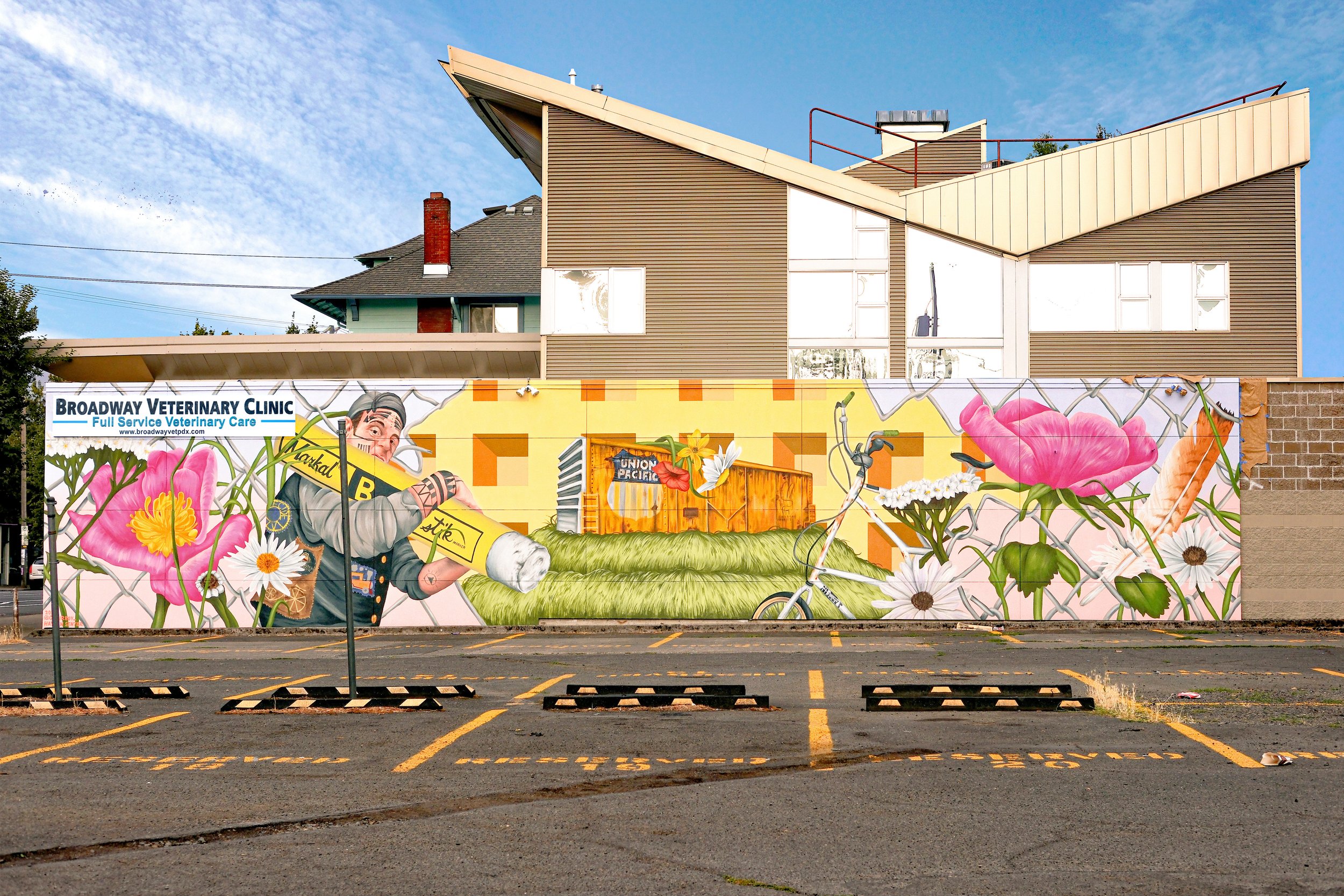The photograph captures a horizontally aligned rectangular image of a multi-storied building and a parking lot in front of it. The building, primarily brown with white cutouts, features a unique roof design that curves inward towards the center. The sky above is clear and blue with a few white, feathery clouds. Dominating the building's facade is a large, colorful mural that reads "Broadway Veterinary Clinic: Full Service Veterinary Care." This mural is adorned with large pink flowers, a man wearing a backward hat and suspenders, holding a gigantic yellow tube resembling toothpaste, a bicycle, and what appears to be a shed or barn atop some hay. In the foreground, the gray asphalt parking lot, marked with various black tar lines to seal cracks, is divided into parking spaces outlined with yellow lines and labeled as reserved. Black concrete barriers are positioned to prevent vehicles from crossing over the spots. Grass peeks through on the right side of the lot, adding a touch of greenery to the scene.